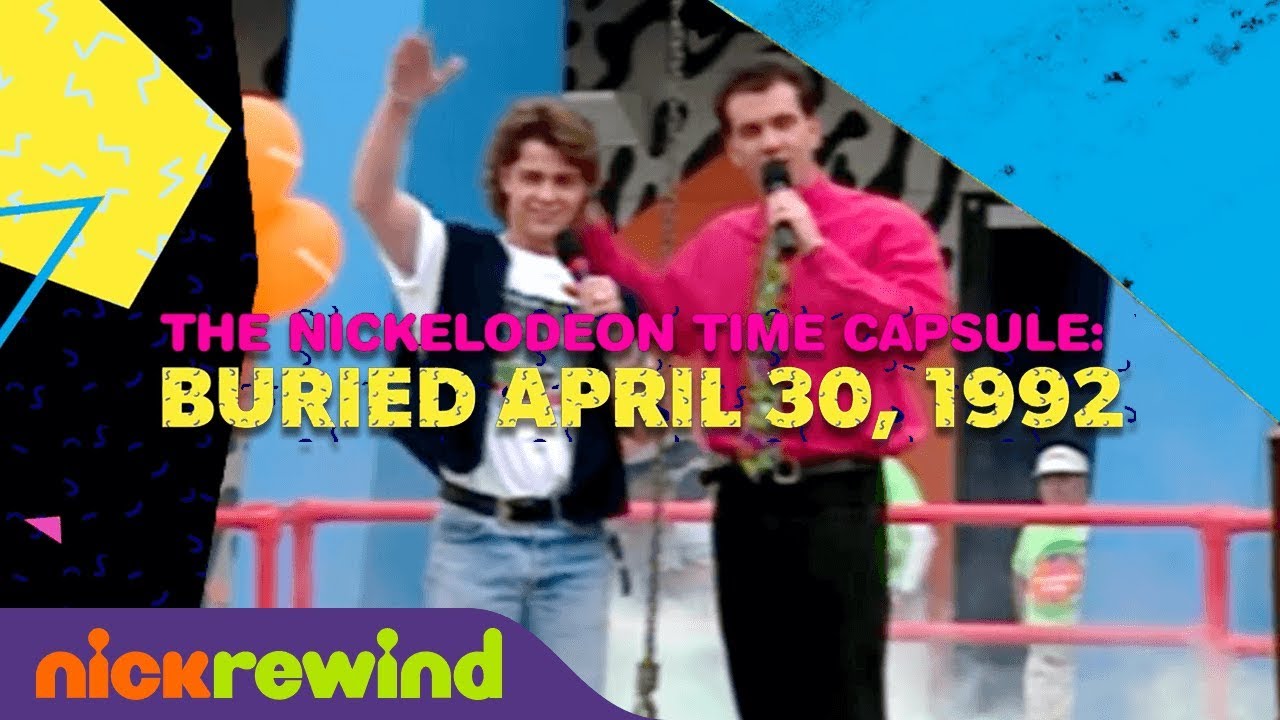The image showcases the ceremonial burial of the Nickelodeon Time Capsule, with prominent text in the middle declaring "Nickelodeon Time Capsule" in pink, and "Buried April 30th, 1992" in yellow right beneath it. On the bottom left, the text "Nick Rewind" is visible, with "Nick" in orange and "Rewind" in yellow. The scene is vibrant, filled with nostalgic, cartoon-like shapes, such as a giant yellow square on the left side adorned with balloons. In the center, a man sporting a black vest, white graphic tee, and blue jeans with a black belt raises his hand, while a man next to him, dressed in a pink shirt with a tie and black pants, holds a microphone and places a supportive hand around the first man's neck. The background features a lively mix of blue hues and zebra print with Nickelodeon employees in green shirts observing. The setting appears to be a screenshot from a video or advertisement commemorating this iconic moment.